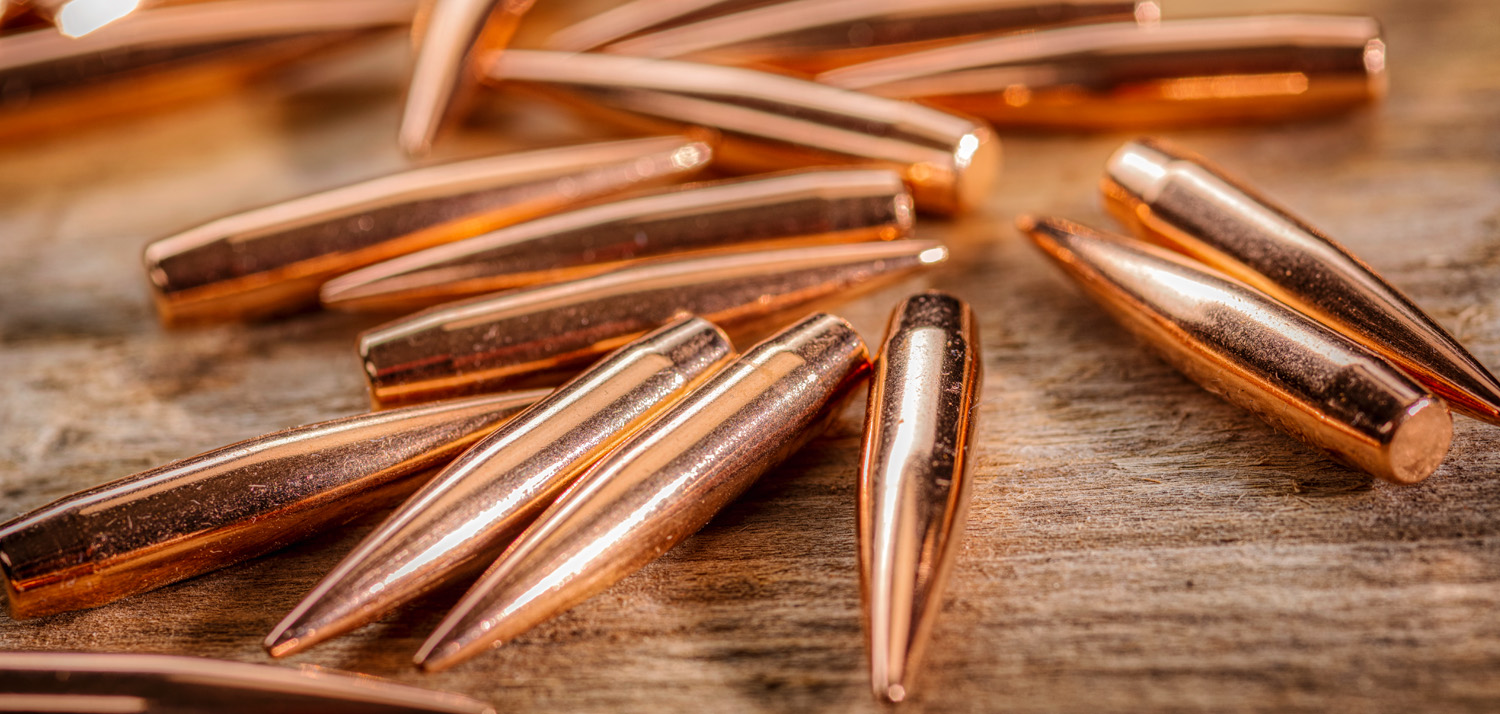The image depicts a scattered arrangement of shiny, brass-cased rifle bullets on a light brown, grained, dusty wooden table. The bullets, torpedo-shaped with tapered, sharp ends, exhibit a rose gold or coppery hue, reflecting light beautifully. The wooden surface contrasts vividly with the smooth, metallic texture of the bullets, highlighting both the artistry of the photograph and the intricate details such as specks of dust and minor scratches on the metal. The bullets are relatively long and flat at both ends, crafted in a seemingly random yet aesthetically compelling arrangement.